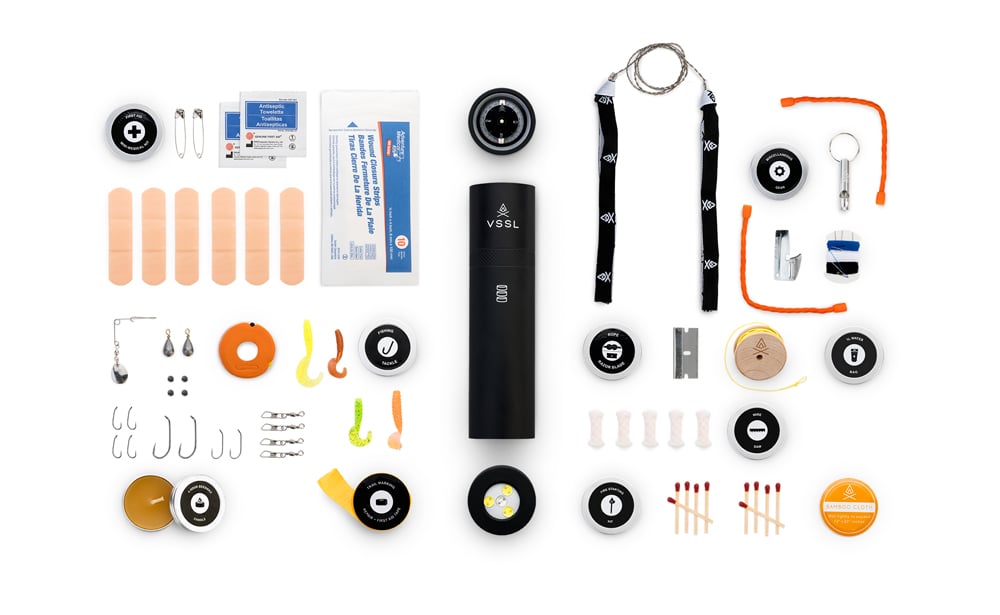The image features a comprehensive emergency kit meticulously arranged against a white background, primarily intended for camping or outdoor activities. At the top left corner, there's a round box marked with a black cross, indicative of its medical contents. Adjacent to this, there are two safety pins and several white packages with blue writing, likely containing assorted bandages. Six band-aids lie unwrapped beside them. Below this medical section, there's a variety of fishing hooks of different sizes, accompanied by fishing bobbers and more hooks.

A small votive candle rests nearby, useful for light or cooking when firewood is unavailable. A compact black case, potentially housing essential tools, sits in the middle of the arrangement, with what appears to be a compass placed above it. Surrounding these items are various fire-starting supplies, including matches and a small orange circle that might be a fire starter.

On the right-hand side, there’s an assortment of useful tools: a razor blade, lengths of wire, and thread with needles. Several black and light brown buttons are scattered throughout, indicating their use for garment repairs or other practical purposes. There's also a carabiner, a piece of orange rope, and some yarn or fiber wire, which could be used for securing or tightening objects. The kit is evidently designed to cover a broad spectrum of emergencies, making it an indispensable resource for any outdoor enthusiast.